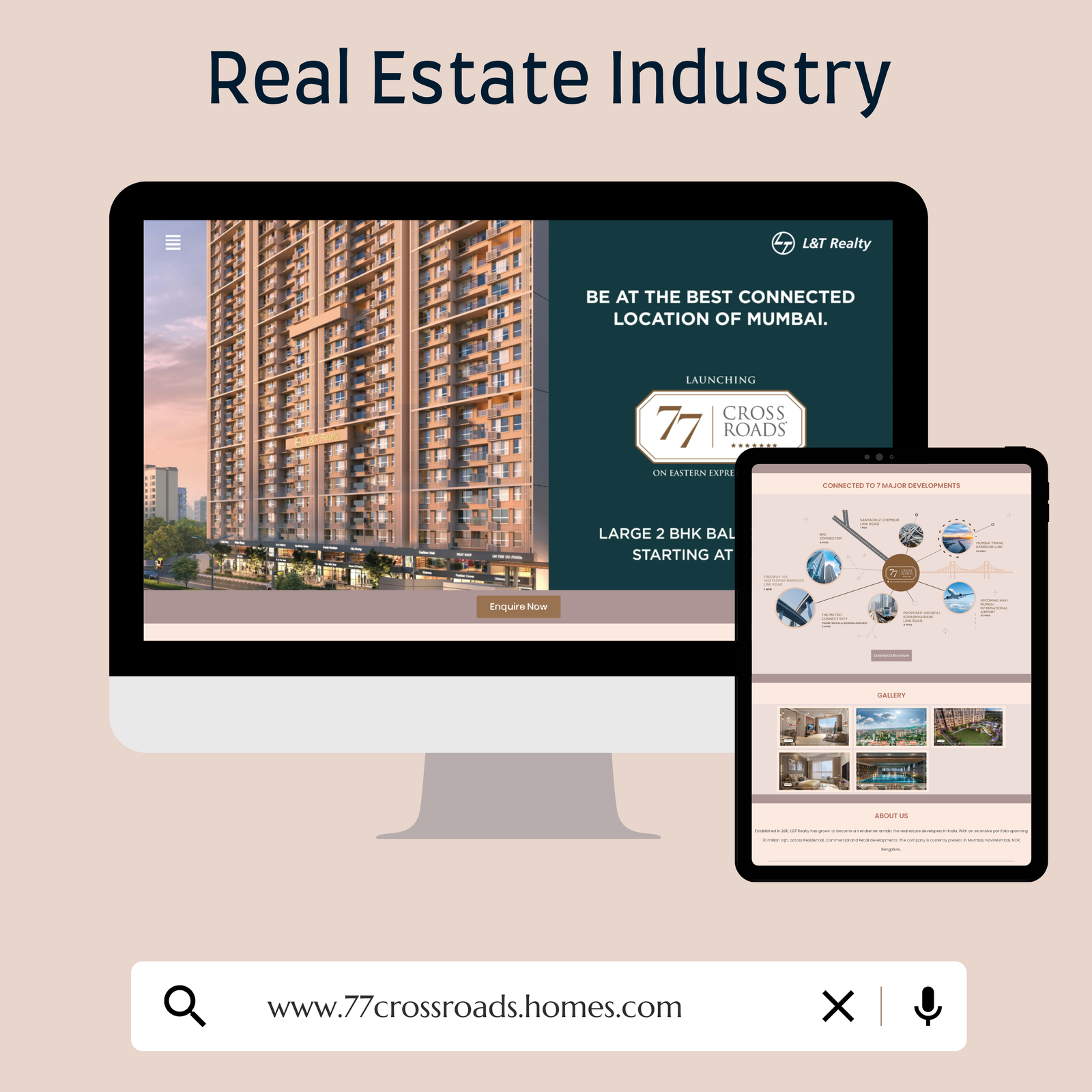In this image, the predominantly black background is accented by gray text at the top, stating "This is the real estate industry." The focal point is a generic-looking iMac with a black bezel, white bottom, and gray stand. Displayed on the iMac screen is a high-resolution image of a tall high-rise building set against a blue sky with scattered clouds. There are also brown buildings in the background and a prominent tan-colored building, resembling a large apartment complex or hotel with numerous windows.

To the right of the iMac, an iPad with a black bezel is shown. On the iMac screen's right side, there's a black tab with a bluish background. At the upper left of this section, white text reads "L&T Realty." Centered below that, additional text states, "Be at the best connected location of Mumbai." Beneath this, a ticket-shaped graphic features black text on a white background stating "77 Crossroads." Further details below this include information about the property, but are partially obscured by the iPad.

On the iPad, barely visible content appears to relate to the 77 Crossroads property. At the image's bottom, a white search bar is visible, featuring a magnifying glass icon on the left and black text that reads "www.77crossroads.homes.com." Adjacent to the search bar are a black 'X' icon and a black microphone icon, prompting users to utilize voice search for inquiries.